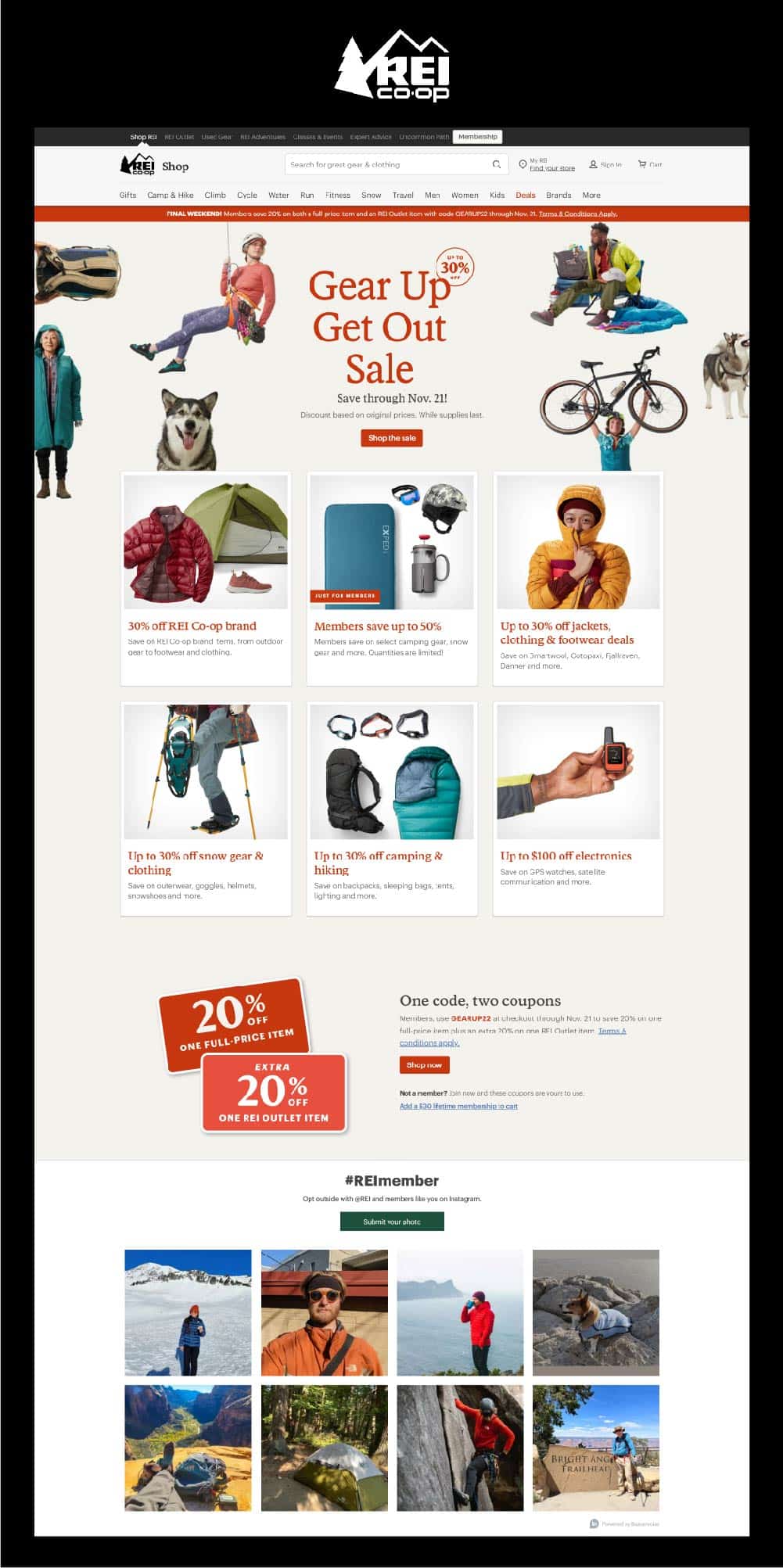This image is a detailed screenshot of the REI Co-op online shopping website. The top of the page features a sleek black bar showcasing a white logo depicting a stylized tree and mountain, with "REI Co-op" written below. Directly beneath, there's a white navigation bar displaying the logo once more alongside a search field equipped with a magnifying glass icon for product searches.

Proceeding downwards, there's a catalog menu bar, though the text is quite small and indistinct. Just below, a prominent red bar with white text grabs attention, followed by a bold red-font announcement stating, "Gear Up, Get Out Sale, Save Through November 25th."

On the right side of the webpage, a dynamic collage of images portrays a man triumphantly lifting a bike, a husky howling towards the sky, and another man comfortably working on his laptop while seated in a lawn chair. To the left of this visual array are the close-up of a husky's head and a man suspended from a rope, adding adventure and activity to the scene.